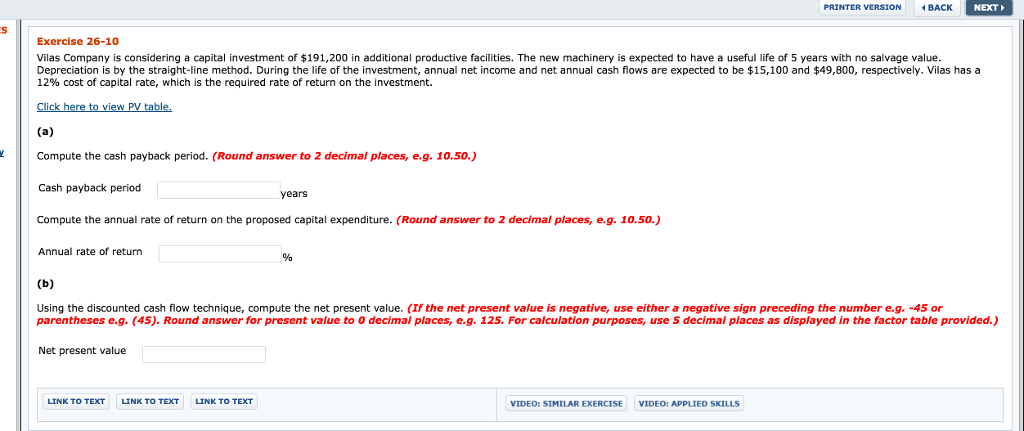This screenshot displays a financial exercise document titled "Exercise 26.10, Phyllis Company is considering a capital investment". The layout presents pages side-by-side, positioned from left to right. On the left-hand side of the visible page, a gray stripe vertically descends, along with a snippet of red text at the top followed by blue text approximately two inches down, indicating the previous page.

In the top right corner, navigation buttons are available: a "Back" button and a "Go Ahead" button, both adjacent to the "Printer Version" option.

The exercise provides detailed instructions and requests calculations for Phyllis Company's potential capital investment in additional productive facilities. Specifically, it asks for the computation of the cashback pay period (presented in years), the annual rate of return, and the net present value. The document also features several "link to text" references and an option to view a similar exercise via video.